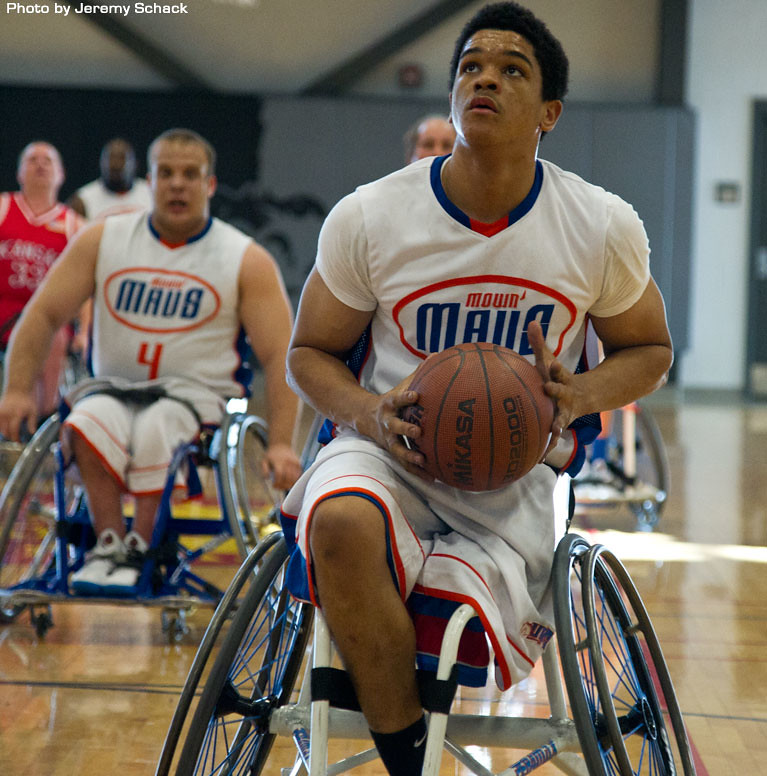This image captures a dynamic moment of wheelchair basketball in an indoor gymnasium with wooden floors. In the foreground, a black adult male, missing his left leg, is poised to shoot a basketball. He wears a predominantly white jersey with red and blue accents and the word "MOUN MAUS" on it, along with matching white shorts with a red trim. His expression is one of intense focus as he looks up towards the hoop. Just behind him to the left, is a white male teammate also in a wheelchair, wearing the same white uniform with red trim and the number four. He appears to be maneuvering his wheelchair forward, perhaps to assist in the play. Further in the background, other players in red and white jerseys are slightly blurred, emphasizing the motion and activity of the game. Some figures, possibly spectators, are visible standing along the sides. The scene is set against a backdrop of gray lockers and white walls, making the competitive spirit of the basketball game the focal point.